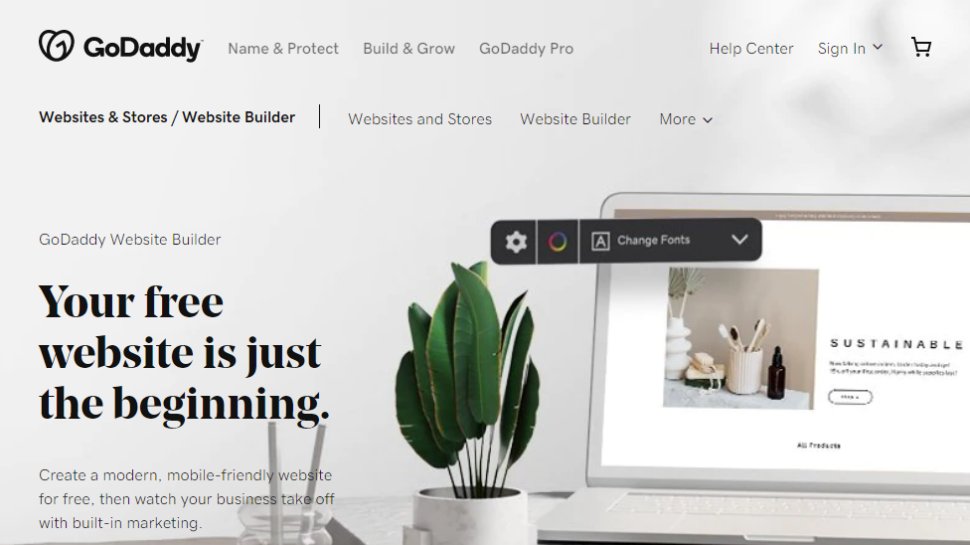A screenshot of the GoDaddy website features its iconic logo in the upper left corner alongside a stylized heart. Adjacent to this, the words "Name and Product, Build and Grow, GoDaddy Pro" are displayed in gray. In the upper right corner, there are links for the "Help Center," a sign-in dropdown, and a black shopping cart icon. Below this navigation bar, the title "Website and Store / Website Builder" appears, accompanied by dropdown menus under "Websites and Store" and "Website Builder," highlighted in gray.

Central to the page, prominently featured in large font, the tagline reads: "Your free website is just the beginning." Directly beneath, it invites users to "Create a Modern Mobile Friendly Website for Free" and promotes its benefits with the line, "Then watch your business take off with built-in marketing."

On the right side of the page, there is an image of a white laptop with a "Sustainable" label on its screen and a green plant in a white pot next to it, set against a white background. Overlaid on this photograph is an interactive element labeled "Change Font" with a dropdown menu, featuring a rainbow-colored circle and a settings icon, offering customization options.